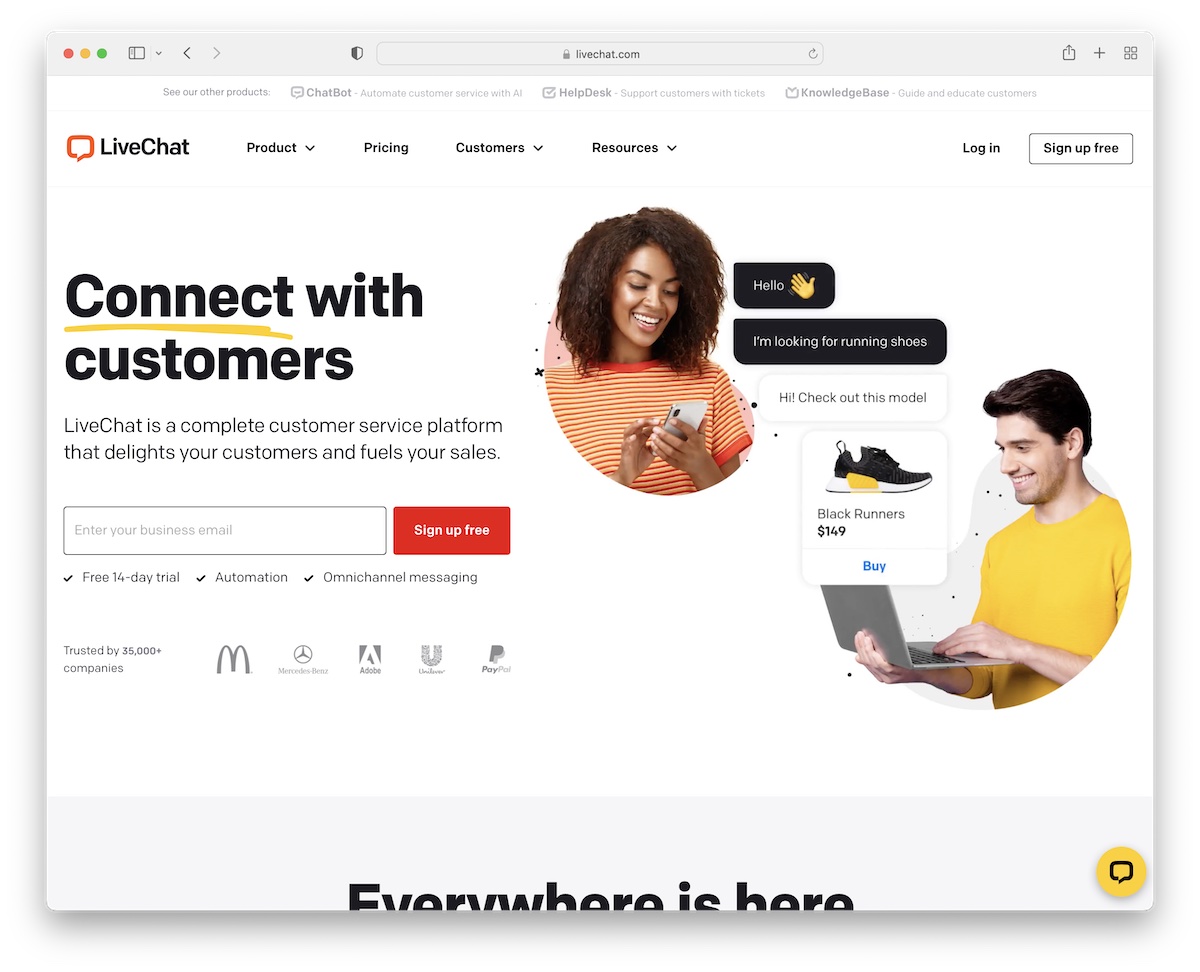Screenshot from LiveChat.com: A comprehensive layout displaying the robust features of LiveChat. At the top of the interface, a header invites users to explore additional products including 'ChatBot' for automating customer service using AI, 'HelpDesk' for supporting customers via tickets, and 'Guide' for educating and steering customers. The navigation bar includes options for 'Live Chat', 'Product', 'Pricing', 'Customers', 'Resources', followed by 'Log In' or 'Sign Up Free'.

On the left side, a prominent section reads "Connect with Customers" with a subheading explaining that LiveChat is a complete customer service platform designed to delight customers and boost sales. This section includes a text box for users to enter their business email and a red 'Sign Up Free' button. Beneath this, several features are highlighted with check marks: 'Free 14-day trial', 'Automation', and 'Omni-channel messaging'.

Further down, it is noted that over 35,000 companies trust LiveChat, with recognizable logos of major brands such as McDonald's, Mercedes-Benz, Adobe, Unilever, and PayPal displayed. 

On the right side of the screenshot, there are images illustrating the chat interface. One shows a woman with dark skin, curly hair, and an orange striped shirt, engaged in a text conversation with a man wearing a yellow long-sleeve t-shirt, with dark hair and holding a laptop. The chat dialogue includes her inquiry, "Hello, I'm looking for running shoes." He responds, "Hi, check out this model," introducing a product description: "Black runners for $149" with a direct purchase option.